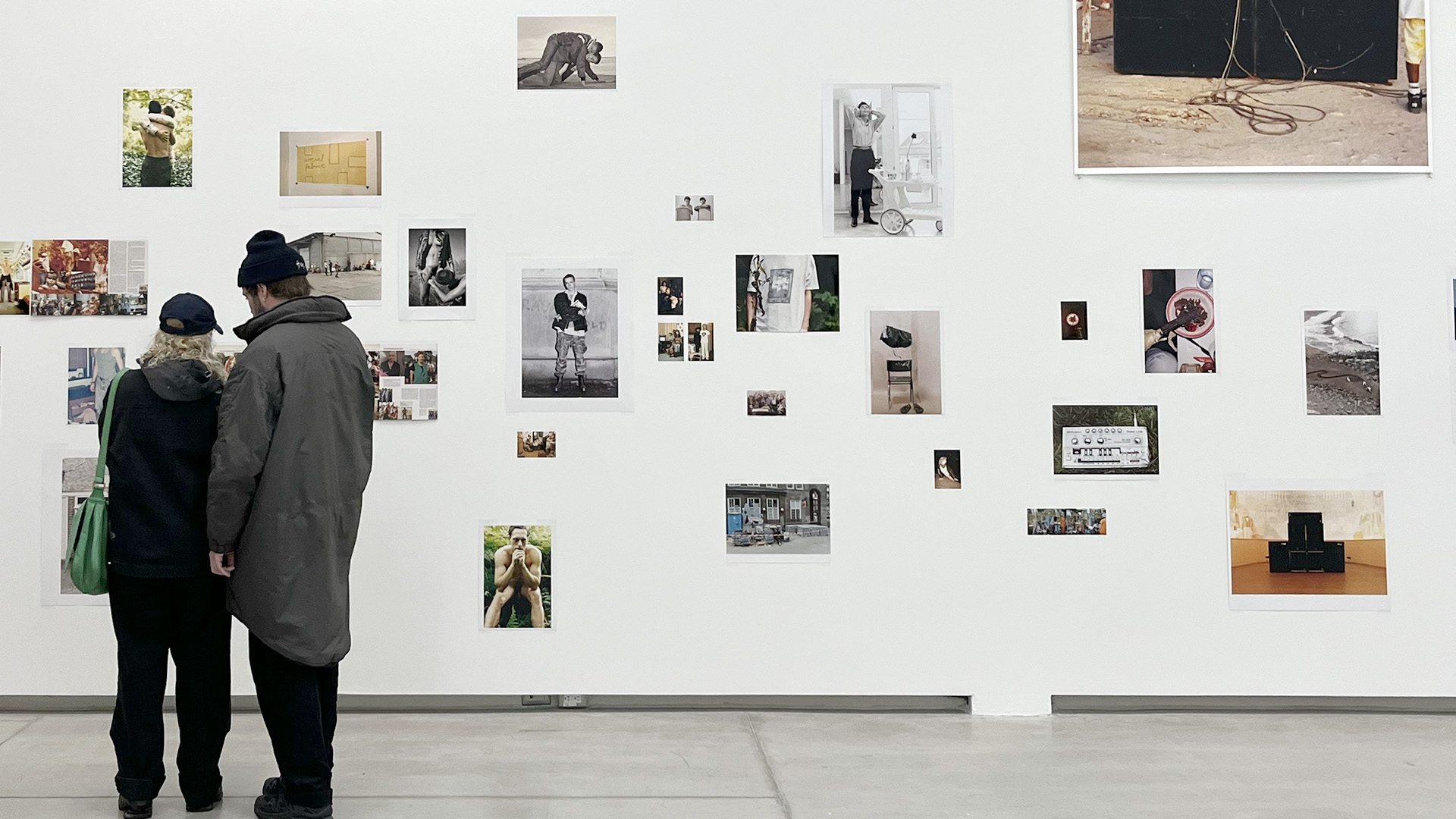In an art museum or gallery with a gray concrete floor, a couple stands closely together, observing an eclectic mix of unframed photographs and magazine articles taped to a large white wall. The woman, with wavy curly gray hair tucked under a black baseball cap, wears a black jacket and black pants, and carries a green handbag. Beside her, the man dons a gray knee-length overcoat, black pants, black shoes, a black wool stocking cap, and a beanie with a pom-pom on top. The displayed images vary from black and white to color, featuring scenes of people, objects, and landscapes, including a man with folded arms, people with shirts off, and still-life compositions of food and personal items. Both individuals are dressed in winter attire, further emphasizing the season. The photos, which seem to capture a wide array of subjects, are randomly arranged across the wall, adding to the casual yet captivating ambiance of the exhibit.